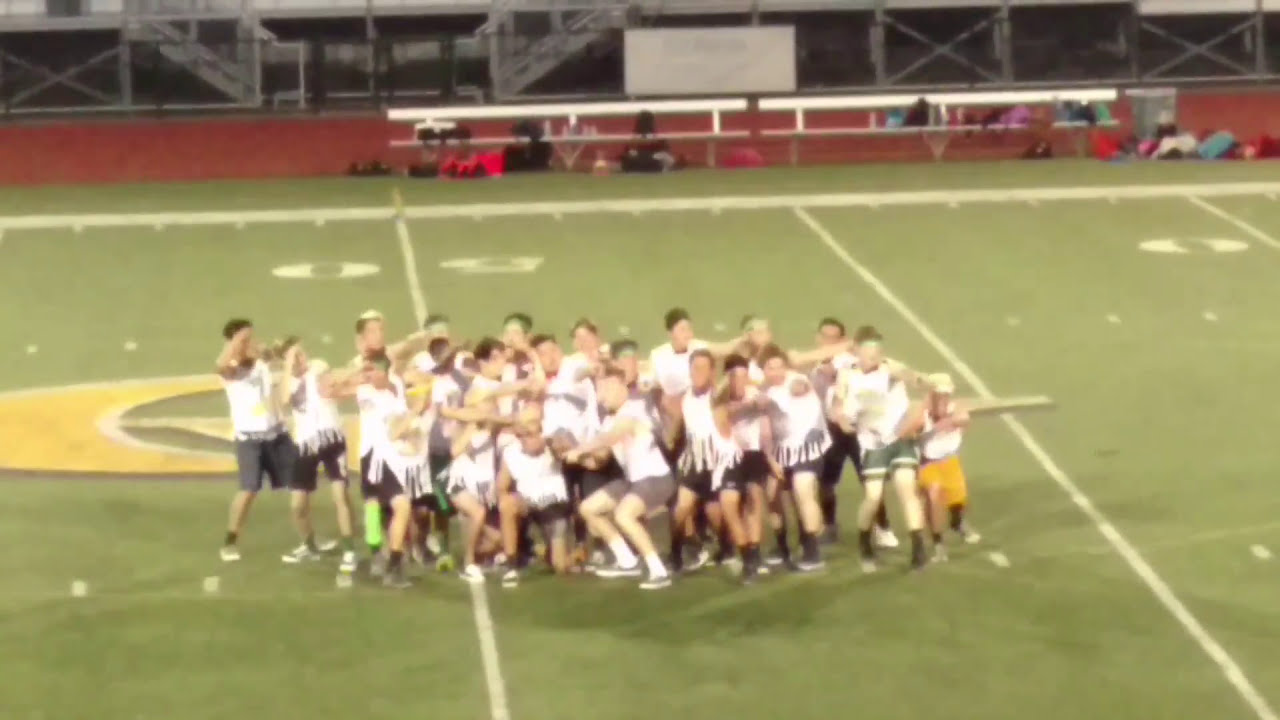This photo captures a lively scene of approximately 20 men, possibly boy dancers or sports players, gathered together on a green field marked with white yard lines and a yellow logo on the left. The group, clad in white t-shirts with frayed edges and white strips, paired with shorts and Vans shoes, is animatedly pointing in various directions, suggesting they are either celebrating or dancing. Their actions convey a sense of recent success or joyful energy. The scene is blurred, making it difficult to discern finer details. In the background, a short reddish-brown wall and a white bench strewn with water bottles and jackets can be seen, reinforcing the notion of a sports venue, possibly a football or soccer field.